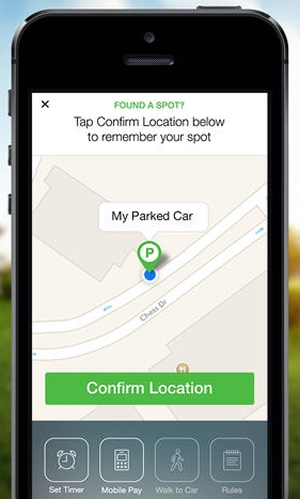The image shows a vertically oriented black cell phone with its screen turned on, set against a backdrop of blurred clouds, sky, and green grass. The phone has three buttons on its left side and one button on its top right corner. Visible on the front are a small hole, presumably for the camera, and the speaker.

The cell phone's screen displays a map, where a road diagonally stretches from the mid-center right to the lower-center left. A green pin is placed on this road. At the top of the screen, there is a white header featuring a black 'X' in the left corner. Below this, in green text, it reads, "Found a Spot." Further down, in black text, the screen instructs, "Tap confirm location below to remember your spot."

Additionally, there is a pin marked with the letter 'P' enclosed in a white circle. Above this pin, in a white box, it says "My Parked Car" in black text. Towards the bottom of the screen, a green button is labeled "Confirm Location."